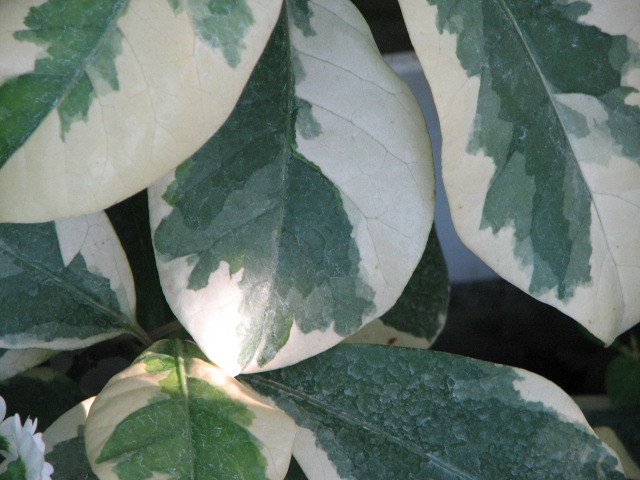The image is a detailed close-up of several large plant leaves, exhibiting a mix of white and green hues. Some leaves are predominantly green, while others have only patches of green, ranging from dark to light tones, with some appearing almost yellowish. Dew or water droplets are visible, adding texture to the image. Among the seven distinct leaves, one stands out with a bubbly texture due to the prominent green cover. In the lower left corner, white flower buds are visible against a dark background, indicating a shaded setting with light breaking through in places. This interplay of light suggests the sun might be rising, illuminating the dew-covered leaves. The image captures the delicate variance in leaf coloration and the subtle beauty of nature's early morning moments.